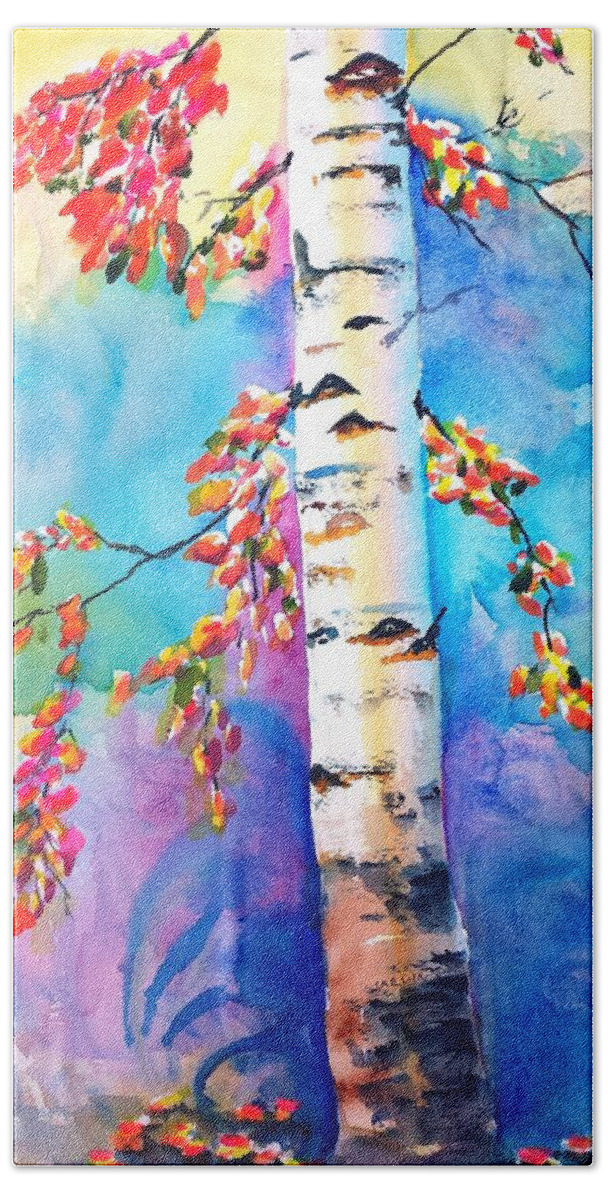A vibrant vertical painting features a striking white birch tree with distinctive black ridges. The tree stands centrally, with its trunk running from the bottom right towards the middle of the artwork. The background is a dynamic blend of pastel hues, transitioning from deep purple at the bottom left, to dark blue, then teal, light blue, and finally pastel yellow at the top. Thin branches extend from the trunk, adorned with a mix of orange, yellow, red, and some pink flowers. At the top left, a larger cluster of flowers adds to the vivid array. Beneath the tree and around its base, smaller patches of red and yellow flowers playfully peek through. The entire image is characterized by textured, broad brushstrokes, suggesting a watercolor medium and creating a beautifully colorful and intricate scene.